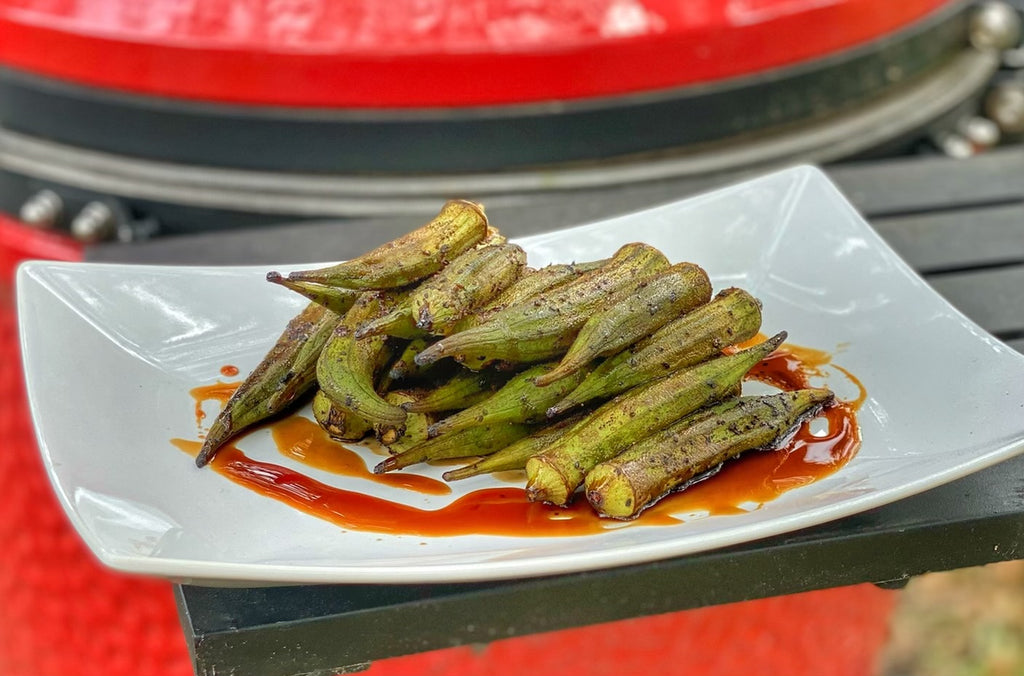The photograph features an outdoor scene, centered around a vibrant red and black grill with an adjacent dark-brown side table. On the table rests a reflective, square-shaped white ceramic plate with elegantly curved tips. The plate features a circular pattern of red sauce – possibly hot sauce – on which lies a generous serving of cooked green okra, likely upwards of 18 pieces. The okra is arranged both side-by-side and stacked atop one another, and is lightly charred with a dusting of an unidentified brown spice. The background hints at a grassy area, suggesting the setting is an outdoor yard. The grill, with its shiny metallic red surface reminiscent of a sleek sports car, stands out against a red surface below, potentially a rug or painted mat, completing the vibrant outdoor culinary setup.